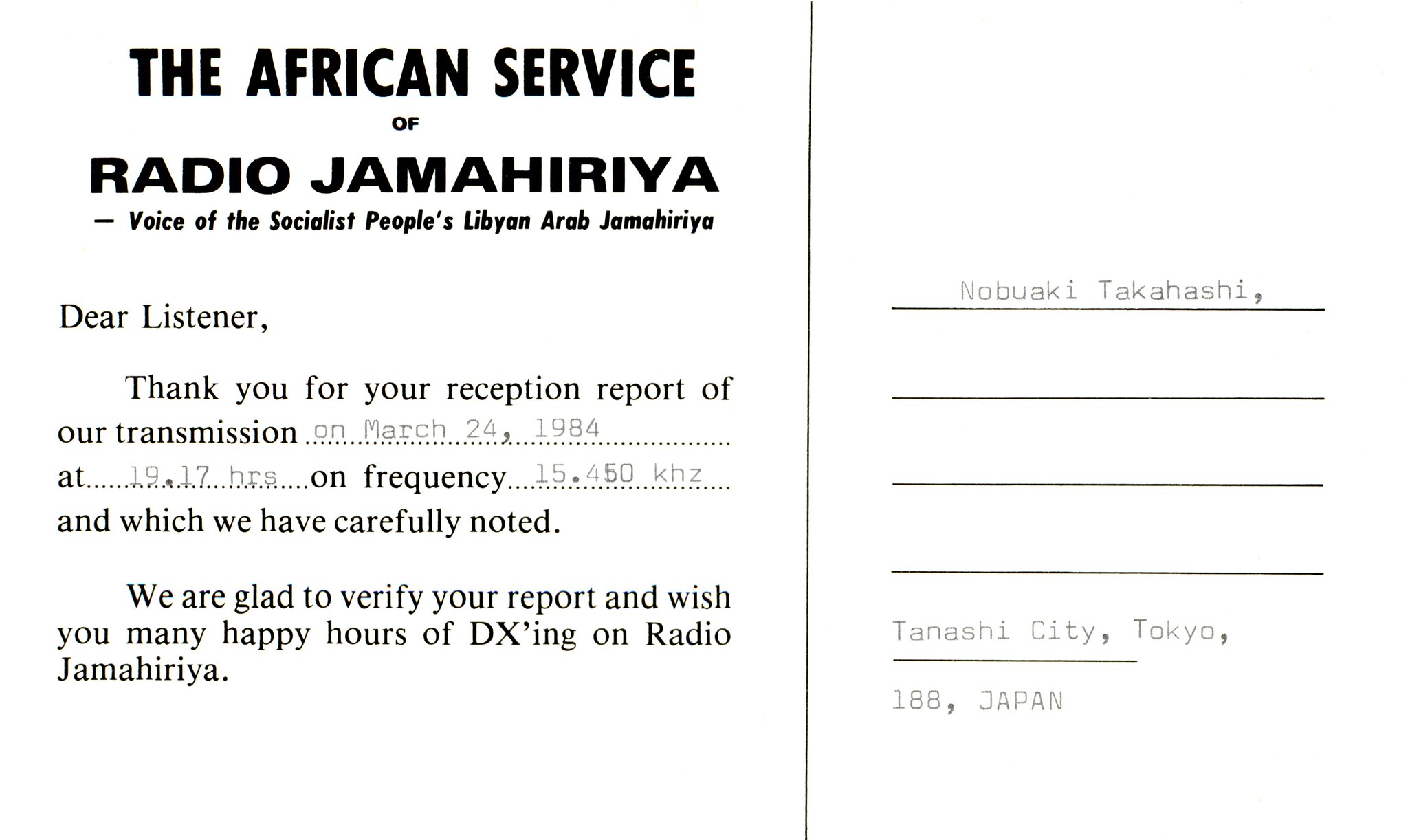The image depicts a postcard-like card divided vertically by a black line. The left side of the card contains a detailed message starting with a header that reads, "The African Service of Radio Jamahiriya, Voice of the Socialist People's Libyan Arab Jamahiriya." Below the header, the text addresses the recipient, stating, "Dear Listener, Thank you for your reception report of our transmission on March 24, 1984, at 19.17 hours on frequency 15.40450 kHz, which we have carefully noted. We are glad to verify your report and wish you many happy hours of DXing on Radio Jamahiriya." 

The right side of the card features the recipient's details: "Nobuaki Takahashi" at the top, followed by the address "Tanashi City, Tokyo, 188, Japan." The background of the card is white, with black text and lines providing structure. Five horizontal lines on the right side organize the text into neat sections, while the left side of the card is dedicated solely to the message.